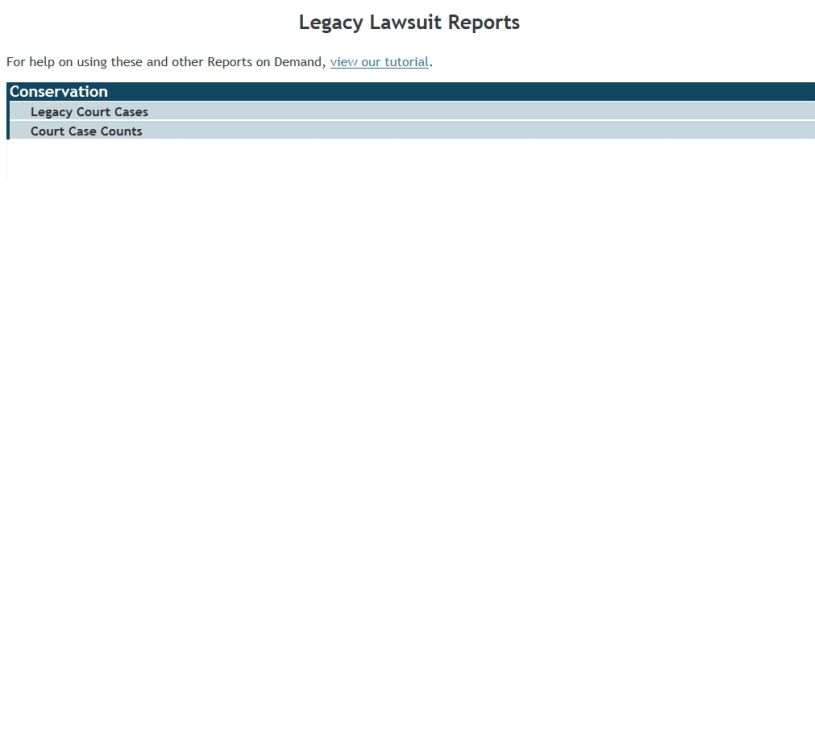The image titled "Legacy Lawsuit Report" features a predominantly black header with the main title in bold, accompanied by smaller black text underneath that reads, "For help on using these or other reports on demand, view our tutorial." The phrase "view our tutorial" is underlined and highlighted in green.

Below the introductory text, a chart is presented, prominently displaying the title "Conservation" in a dark green box with white text. The chart itself is composed of alternating light gray and white lines, creating a clear separation between data fields. The primary categories listed within the chart are "Legacy Court Cases" and "Court Case Counts."

Despite the detailed layout, the image occupies only the upper portion of the available space, leaving a substantial white area below. There is also a note indicating, "Please talk for 90 seconds," directed at the users or participants, but it does not seem to affect the image’s content. The image does not expand upon reloading and appears to be a narrow strip within a larger blank area, suggesting either a display error or that the image was intentionally designed with significant white space.

The overall color scheme of the image includes dark green, light green, white, and black, which harmonize well with the subject matter of legacy lawsuit reports. The design focus is on providing information regarding court cases and their respective counts, though the layout leaves some ambiguity regarding the full utilization of space.